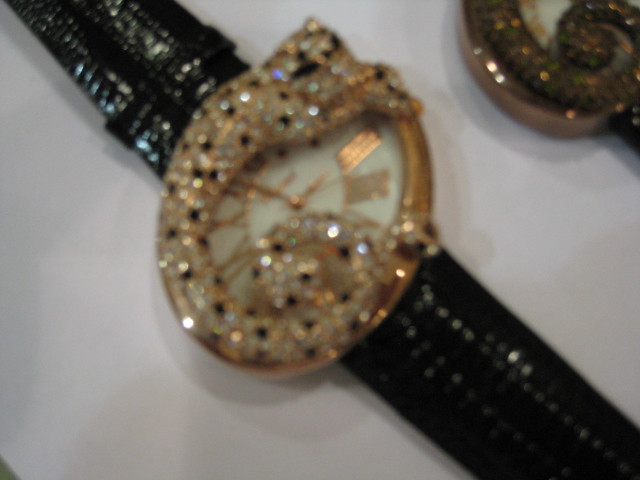The image captures a close-up of a wristwatch laid out on a white surface, illuminated from the top to create a subtle shadow effect. The black leather strap, which appears to have a snakeskin or crocodile texture, elegantly loops around the wrist. The watch's face is encased in a gold trim, featuring a striking design composed of shiny little diamonds and black stones. The background of the clock face is either white or gold, embellished with an intricate arrangement that resembles a leopard or cheetah pattern. The watch's face is oval-shaped and displays time in gold Roman numerals, although it appears slightly tilted or upside down. Notably, there is a detailed depiction of a cat, crafted from the diamond and stone accents, resting on the exterior of the watch face. The watch hands—hour, minute, and second—are also made of gold, completing the luxurious and complex design.